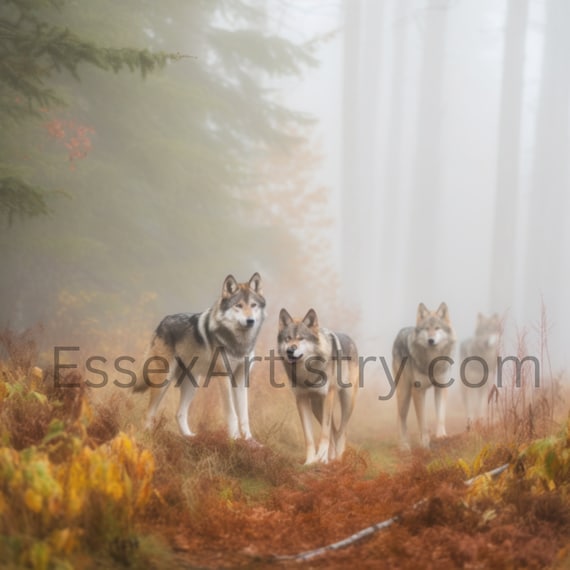In this detailed and atmospheric photograph taken by EssexArtistry.com, we see a mesmerizing scene of a wolf pack within a fog-cloaked forest. The dense fog obscures much of the background, lending an ethereal quality to the image. Four to six wolves, predominantly black, brown, and white in color, are calmly standing and facing the camera, exuding a majestic presence. Their fur is a striking mix of blacks on their backs, browns toward their legs, and whites around their noses and undersides. The forest floor is strewn with twigs, moss, and yellowish-brown grass, hinting at the transition between seasons, underscored by the amber hues of fallen leaves and scattered branches. Towering coniferous trees surround the pack, with a hint of green from some lingering leaves and a bit of brown from strands of bark. The watermark "EssexArtistry.com" in dark gray letters can be seen towards the bottom of the image, subtly blending into the foggy, tranquil atmosphere.